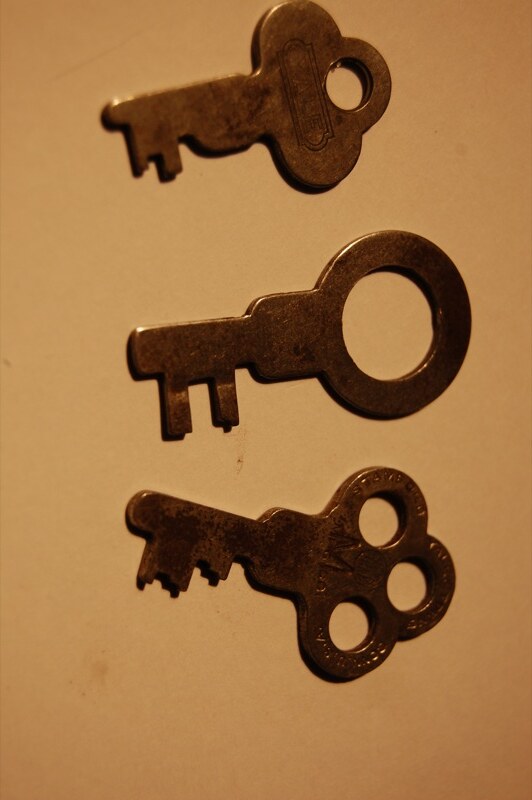This image showcases a close-up of three horizontally aligned, old-fashioned brass keys against a light beige background, possibly a table, countertop, or wall, which appears slightly dirty with little specks. The keys' key portions are on the left, and their handles are on the right. Each key varies in design and has a distinctive patina, indicating age. The top key, which has a brownish hue, features an undecipherable engraved plaque and a circle punch-out on the right. The middle key has a larger, single circle punch-out with two small square notches. The bottom key, which has "M" engraved along with other unreadable text, displays three circular holes and a jagged edge on the left side. These unique keys likely correspond to different types of locks, suggesting various purposes and historical significance.